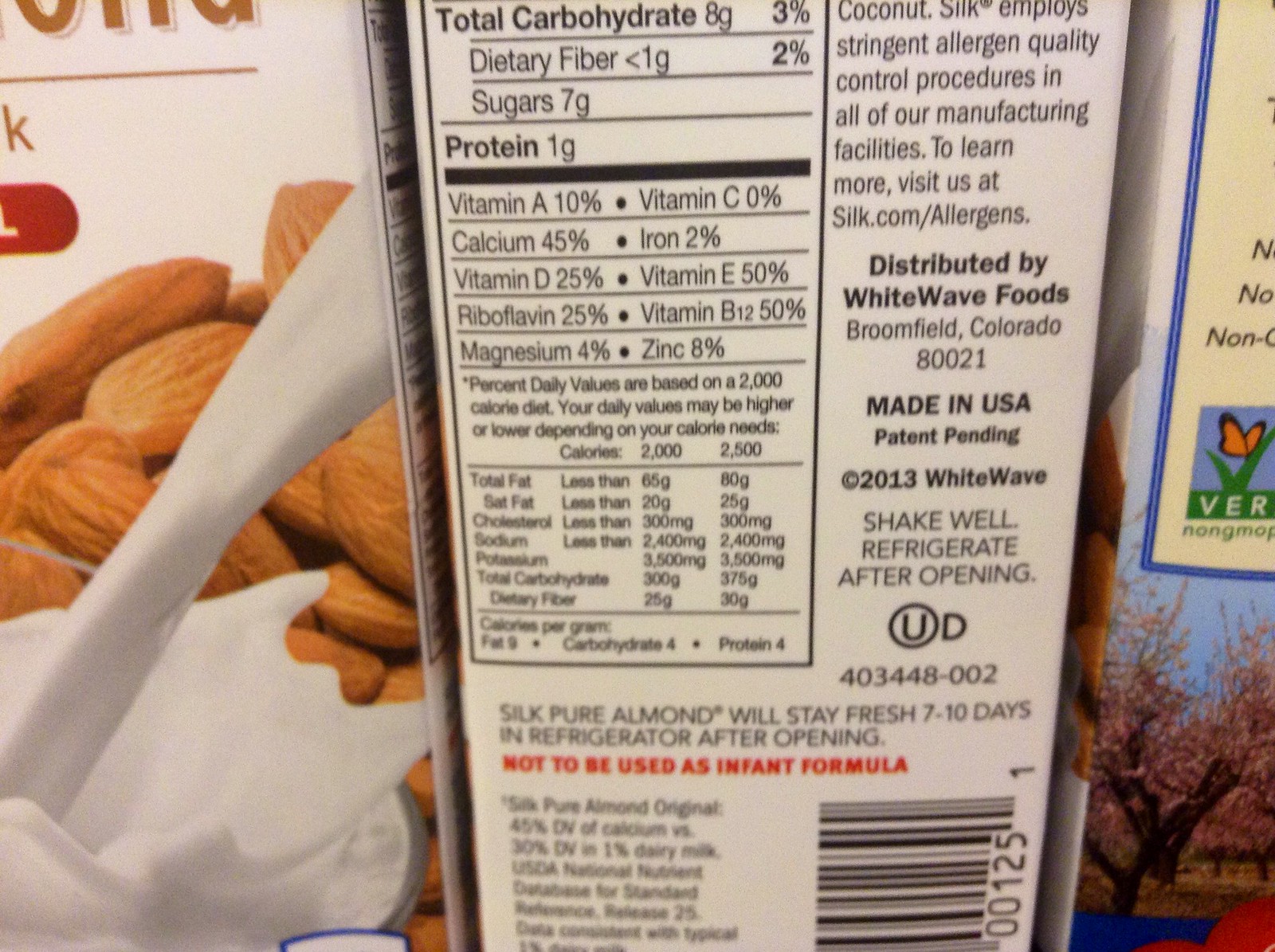This photograph captures a detailed view of the side of a white container, prominently featuring various sections of text and graphics. In the upper left-hand corner, there is a partially visible nutrition information box starting with the bolded text "Total Carbohydrate 8G" and "3%" beside it. Adjacent to the nutrition box is a section of black text, followed by information indicating that the product is distributed by White Wave Foods.

At the bottom right, the top part of a barcode is visible. Centrally positioned below the nutrition information, there is an area of black text that includes a bolded red warning stating, "Not to be used as infant formula." Directly below this warning, on the left, there is additional small white text.

To the left side of this container, another white carton is slightly visible, featuring some cut-off brown text at the top. This second carton also displays an image of milk being poured, with a stream of milk and brown nuts in the background. The detailed arrangement of elements provides important information as well as visual cues about the product's content and intended use.